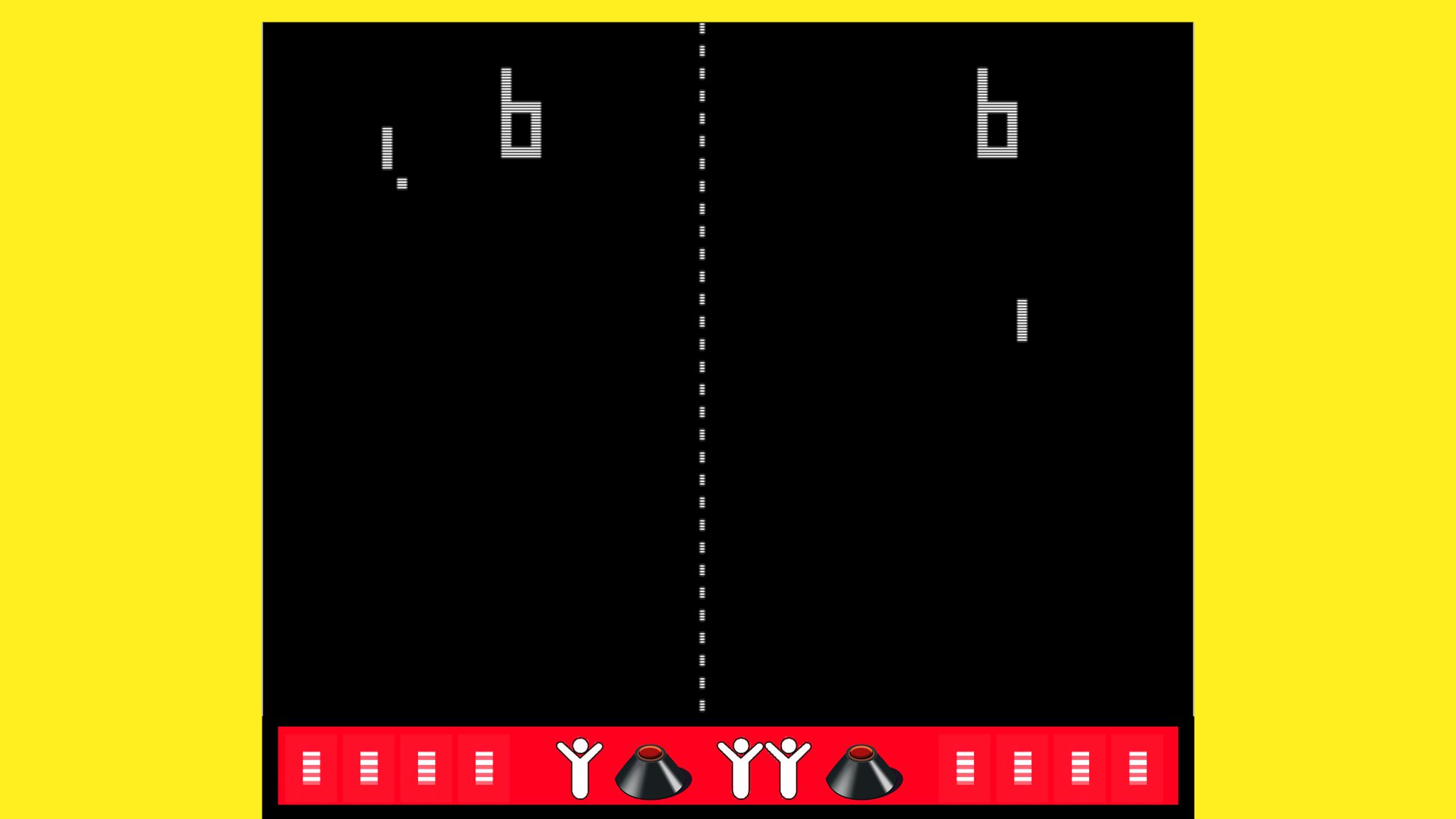This image appears to be a screenshot from a minimalist video game. The image is presented in a rectangular format that is wider than it is tall, with a vivid bright yellow background framing the central game screen. The main gameplay area is a black square situated in the center of the image. A white dashed line traverses the black square vertically, dividing it into two equal halves.

On both sides of this dashed line, within the black square, there are simplistic geometric shapes: on the left side, a small rectangle, a small square, and a shape resembling the number six. The right side mirrors these shapes with identical positioning and form.

At the bottom of the image runs a horizontal red bar, populated by a variety of icons. These icons include different rectangles, stick figures, and shapes that resemble volcanoes, adding an element of intrigue and hinting at possible game functionalities or levels. The overall scene is visually striking due to its contrast between bright yellow and deep black, and it hints at a game that relies on simple yet engaging visual elements.